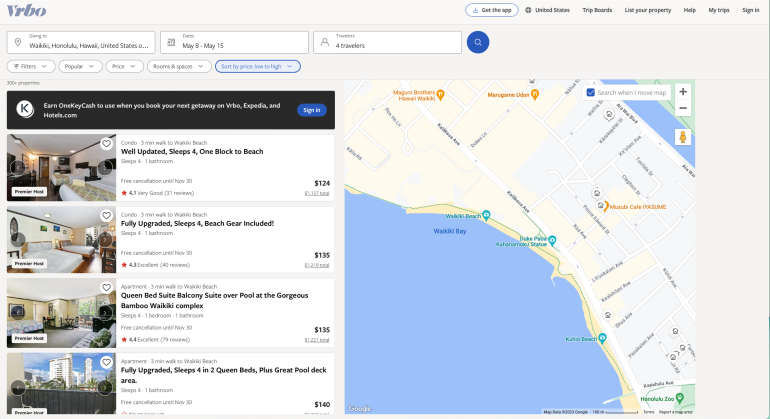This web page from the Verbal VRBO website features a detailed display of various hotel rooms along with their specific locations. At the top, there are three search boxes, the exact labels for which are unclear. These search fields are followed by a row of seven tabs, which likely serve as navigation or filter options. Below the search boxes are additional filter tabs, four in total, each equipped with drop-down arrows for more specific selections.

The main section showcases four prominent images of hotel rooms:
1. The first room image includes a caption that reads "Well-updated, sleeps 4, one block to the beach."
2. The second image highlights a "Fully upgraded, sleeps 4, beach gear included, queen bed suite, balcony suite." 
3. The third image description, though partially unclear, mentions "suite, balcony suite, and gorgeous bamboo Waikiki."
4. The fourth and final room image indicates "Fully upgraded, sleeps 4, two queen beds plus great pool deck areas."

On the right side of the webpage, there's an interactive map that pinpoints the exact locations of these hotels, represented by location icons. Additional nearby accommodations are also marked, assisting users in selecting the best location for their stay.